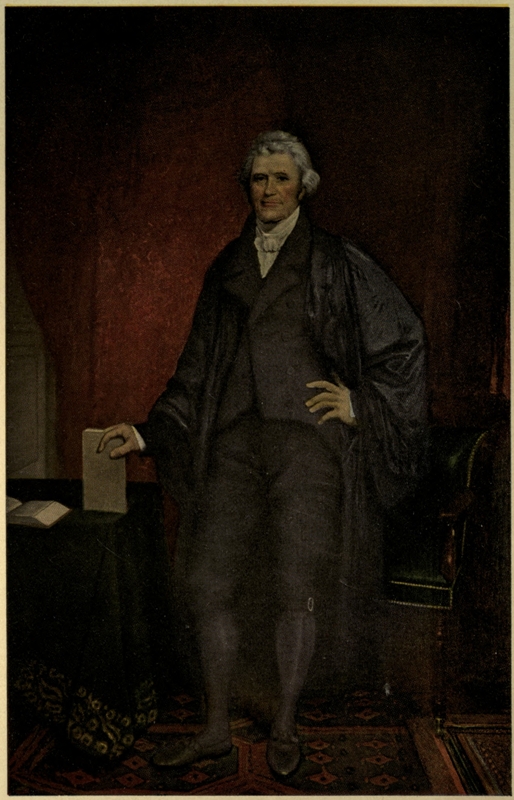This painting depicts a prominent man from the colonial era, possibly a figure like Thomas Jefferson. He stands tall, looking directly at the viewer with fair skin, rosy cheeks, and grayish-white hair styled in curls. He is dressed in a formal black outfit comprising a vest, tight knee-length pantaloons, stockings, shoes, and a long overcoat reminiscent of a judge's robe. His attire includes a white ruffled shirt that reaches up to his neck. 

In his right hand, he holds a book vertically, which rests on a dark wooden desk draped with a green cloth, while his left hand is placed on his waist. Another open book lies beside the one he is holding. The background features a dark red, almost clay-like wall with shadows, adding to the depth of the image. Additionally, a black chair with dark wood, subtly outlined, can be seen behind him. He stands on a rug with dark tones, completing the elegant and historical setting of this detailed colonial painting.